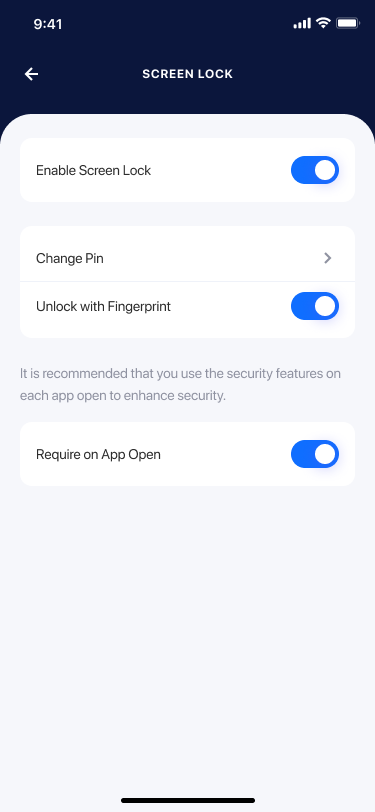This is a detailed caption of the screenshot: 

The image captures a smartphone screenshot featuring a black border. At the top left corner, the timestamp reads "9:41." To the right of the timestamp, there is a Wi-Fi icon indicating a strong signal, and a battery icon showing high battery power. Below the status icons, a left-facing arrow is visible on the far left, positioned next to the words "Screen Lock" centered at the top.

Within the body of the screenshot, the first option displayed is "Enable screen lock," which is toggled on. The next option, "Change PIN," is listed with a right-facing arrow to its right. Below that, "Unlock with fingerprint" is shown, with the toggle also turned on.

Further down, a recommendation: "It is recommended that you use the security features on each app to enhance security" is provided. Another setting, "Require on app open," is listed beneath the recommendation and is toggled on.

At the very bottom of the screenshot is a solid black line representing the home button. This screenshot appears to depict a settings page for the screen lock feature on a smartphone, where various security options such as enabling or disabling screen lock, unlocking the phone with a fingerprint, and requiring screen lock on app open can be managed.